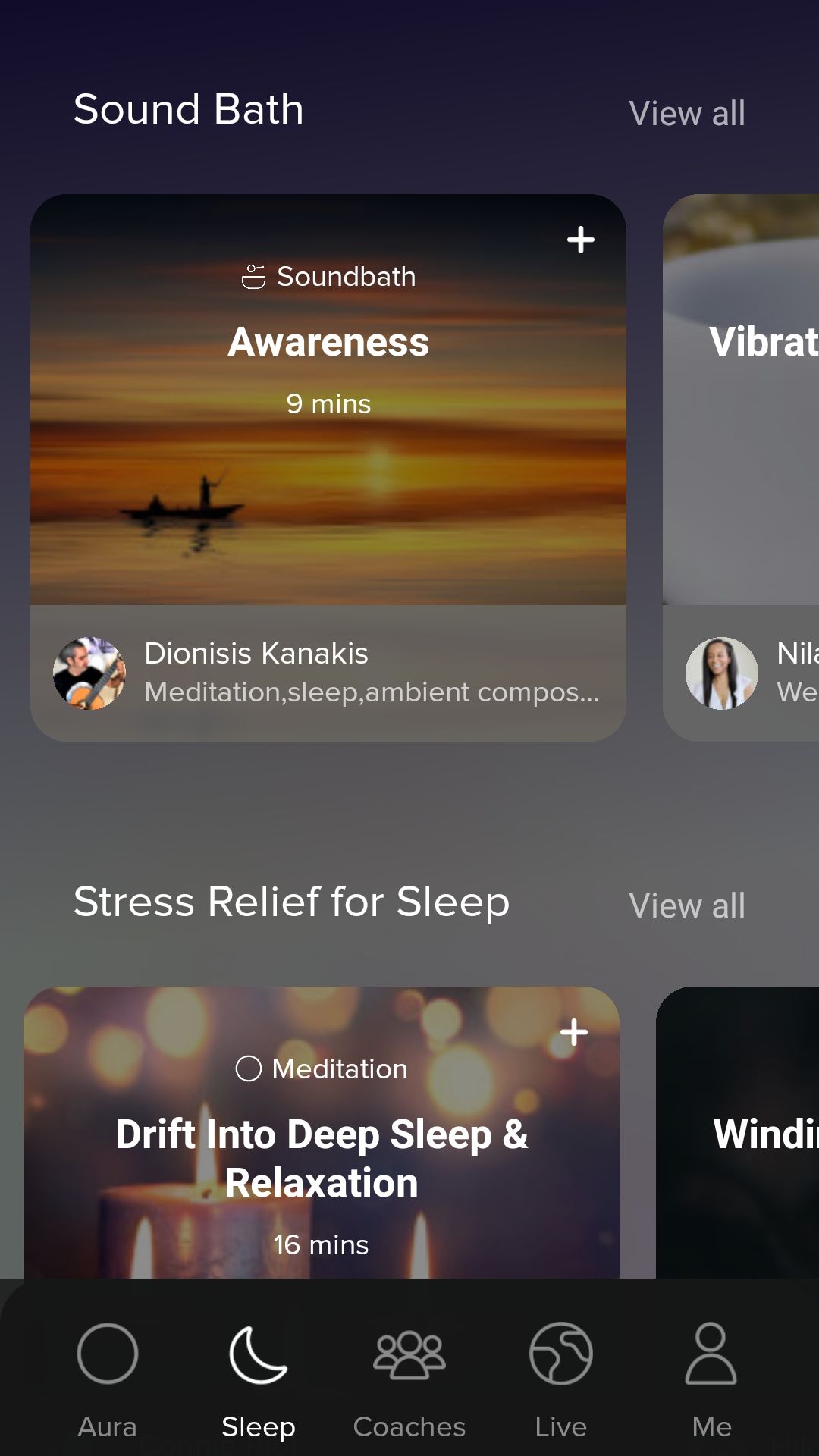This screenshot captures the interface of a meditation app on a mobile phone. The app features several tabs at the bottom of the screen: "Aura" (represented by a circle icon), "Sleep" (marked with a crescent moon icon), "Coaches" (indicated by simplistic profile icons), "Live" (featuring a world icon), and "Me" (displayed with a single profile icon). The currently selected tab is "Sleep."

At the top of the Sleep tab, the section "SoundBath" is highlighted with an option to "View All." Featured prominently in this section is a meditation titled "SoundBath Awareness" by Dionysius Kanakis, described as a "9-Minute Meditation" under the categories "Meditation, Sleep, Ambient, Compose." Accompanying this meditation is a serene image of a canoe on water during a sunset.

Further down, there's another section titled "Stress Relief for Sleep" with an option to "View All." One of the listed meditations here is "Meditation Drift into Deep Sleep and Relaxation," which lasts 16 minutes. The background for this meditation shows an image of candles and softly-focused points of light. Additional meditations are partially visible, cut off along the right side of the screen.